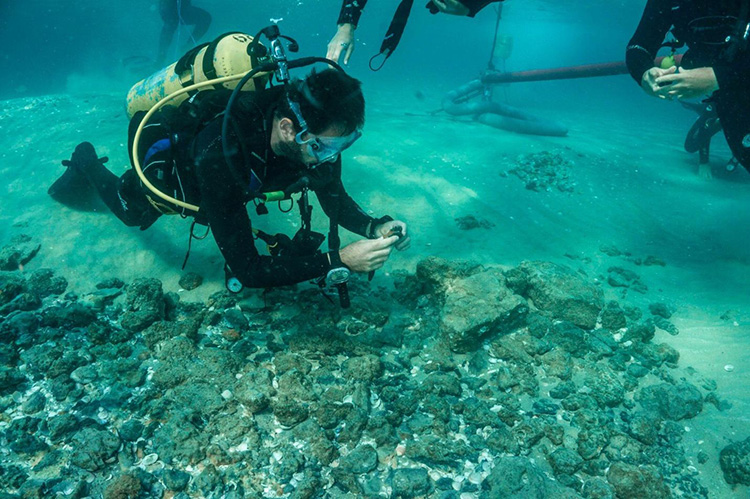This underwater photograph, approximately six by four inches in size, showcases a group of scuba divers exploring a bright blue and clear aquatic environment. The foreground features a man, likely in his 30s or 40s, with dark hair and light brown skin, identifiable by his yellow oxygen tank and black scuba suit. He is intently examining an object, possibly a stone or coral, that he has picked up from a rocky section of the seabed. Surrounding him, the seabed transitions from a rough, rocky terrain to a smoother, sandy surface, both imbued with a bluish-green hue. To his right, the partial figure of another diver is visible, marked by hands and arms, while in the background, additional divers can be seen: one with clasped hands and another's legs faintly discernible. A long hose extends from the upper right corner towards the center, and a hand reaches down from above, likely from another diver. The divers are equipped with black scuba gear, including masks and yellow tanks, and some appear to be documenting the underwater landscape, capturing images of the rocky and sandy seabed.